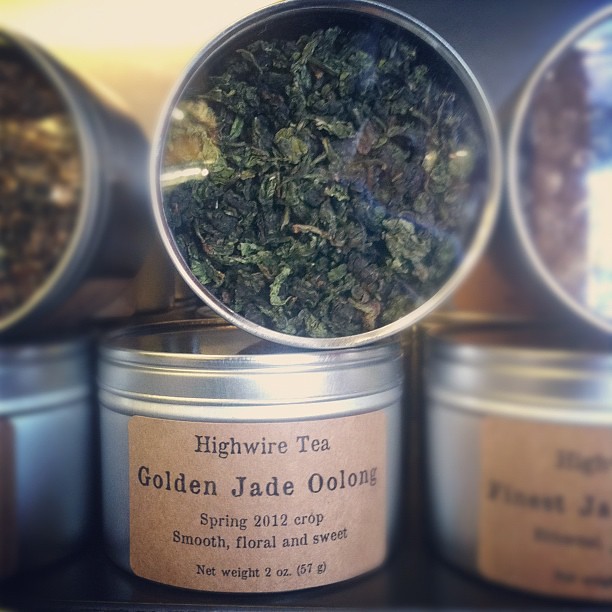The photograph showcases a selection of three stainless steel canisters of tea, neatly stacked with one prominently displayed on a wooden surface. The central canister features a detailed label that reads "High Wire Tea, Golden Jade Oolong, Spring 2012 Crop, Smooth, Floral, and Sweet, Net Weight 2 ounces (57 grams)." This canister's lid, made of clear plastic, allows a view of the dark and light green loose tea leaves inside. The two flanking canisters are slightly blurred but visibly showcase their own distinct colors; the one on the left has a yellowish-brown hue, while the one on the right exhibits a grayish-brown tint. The canisters above the main ones display their contents through transparent tops, providing further insight into the variety of tea leaves within. The arrangement highlights the central canister's vivid green tea leaves, presumably the Golden Jade Oolong, creating a visually appealing and informative display of the tea collection.